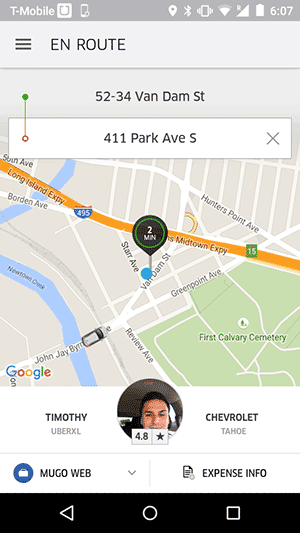The vertically rectangular image is a cell phone screenshot. At the top, a medium gray horizontal banner displays "T-Mobile" on the left side, while the right side shows various status icons including location, Bluetooth, Vibrate, Wi-Fi, signal strength, and battery level. The time reads 6:07.

Directly below this banner, "Enroute" is visible, followed by the route details: from "52-34 Van Dam Street" to "411 Park Avenue South." The image also features a residential map with a pinpoint marker indicating "2 minutes."

Toward the center, an icon representing the driver is shown with a 4.8-star rating. To the left of this icon, the driver's name and service type are listed: "Timothy, UberXL." To the right, the vehicle information is noted: "Chevrolet Tahoe." Below this, there are options labeled "Manage Trip" and "Expense Info."